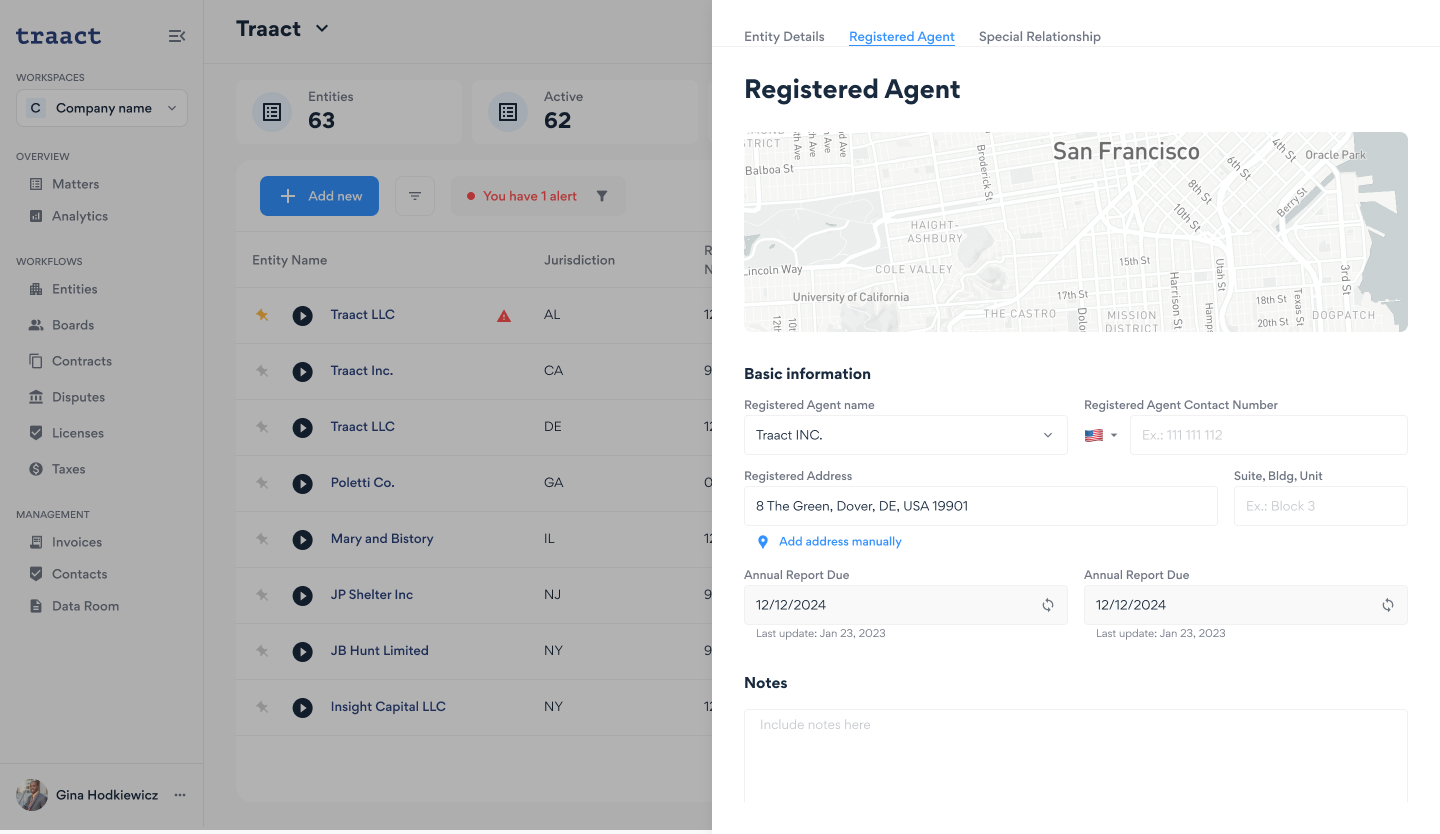The image depicts a screenshot of a web interface on a computer screen, associated with a website or application named "Tracked Website or App." The background of the interface is predominantly white, featuring text in black and blue. 

On the left half of the screen, various elements are displayed:
- The website's name "Tracked Website or App."
- The interface includes textual elements such as "Entities, 63," "Active, 62," and "Add New," with "1 Alert" prominently displayed in red text.
- A menu section features options like "Company Name," "Analytics," "Metas," "Workflow," and "Management."

The right half of the screen has a continuation of the white background and contains:
- Sections titled "Entry Details," "Registered Agent," and "Special Relationship," with "Registered Agent" highlighted in blue and underlined, while the other sections are in grey.
- A map, presumably of San Francisco, accompanies the "Registered Agent" section.
- Additional sub-sections include "Basic Information," an address field, a report section, and an area for notes.